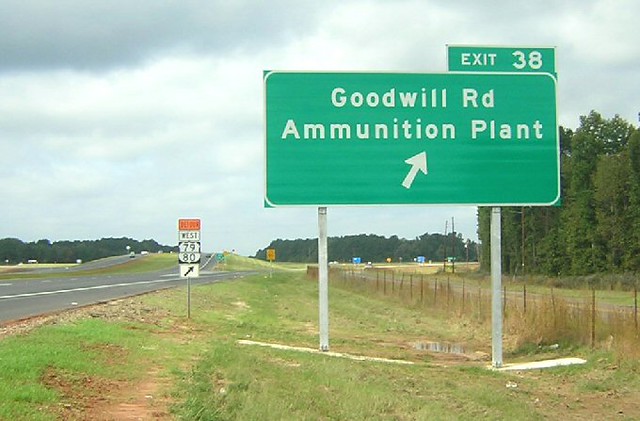This detailed image depicts a segment of a highway marked by prominent signage. The central feature is a large green highway sign, displaying in bold white letters "Exit 38 Goodwill Road Ammunition Plant," accompanied by a rightward-pointing arrow. Adjacent to this green sign stands a highway marker featuring the numbers "79" and "80" within a white shield set against a black background, also directing rightward. The road itself extends straight ahead, with a visible exit branching off to the right. Adding to the scene, a lesser sign in orange and white, marked "Detour West" beside the highway shield symbols and an arrow, provides additional navigational information. The roadside includes a green grassy shoulder, patches of red dirt, and a faintly visible fence. The landscape is bordered by multiple lines of trees, both in the foreground and along the horizon, and the sky overhead is mostly clouded. This spectrum of elements—highway, signs, natural surroundings, and weather—come together to create a comprehensive snapshot of this highway exit environment.